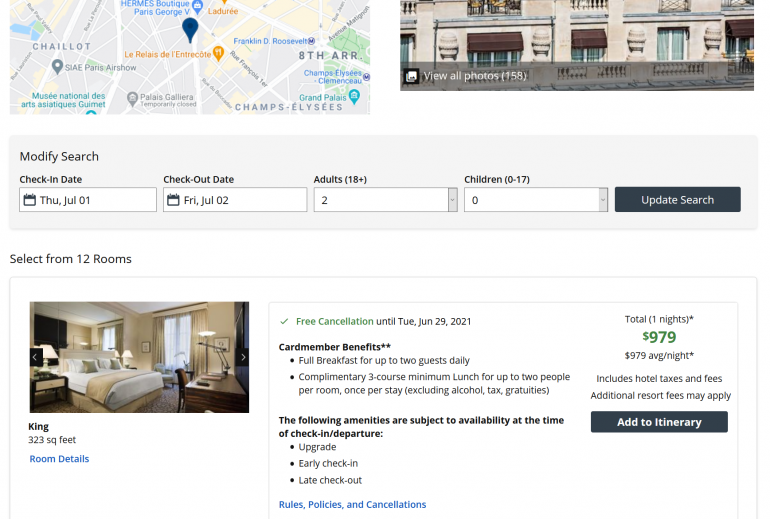This screenshot showcases a search for a hotel room in Paris, with a detailed map highlighting landmarks such as the Champs-Élysées and Palais Galliera in the upper left corner. In the upper right, a horizontal image displays a hotel adorned with a brown awning. Central to the image is a gray search modification box displaying criteria such as check-in date (Thursday, July 1st), check-out date (Friday, July 2nd), 2 adults, and no children, with an 'Update Search' button to the right.

Below this, a large rectangle features comprehensive details about a specific hotel room. The left side presents an image of a spacious room with tan walls and a large, elegant King-sized bed, indicating 323 square feet of space. In the right part of this section, the price for one night is prominently displayed as $979, along with a note about free cancellation. Additional information is also mentioned, and a 'Add to Itinerary' button is available at the bottom right for booking the room.